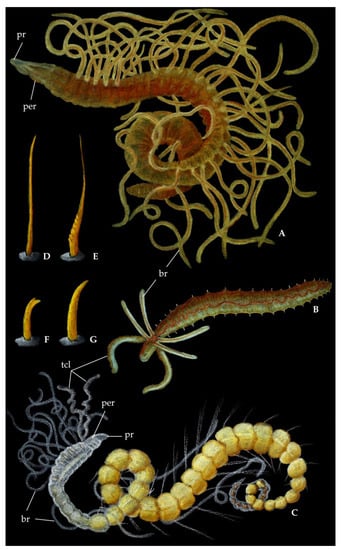This detailed poster, set against a solid black background, depicts three distinct sea creature-like organisms, each occupying its own section from top to bottom. At the top, a dark orange-red creature, resembling a worm, is densely surrounded by tentacle-like appendages that look like tangled spaghetti. These appendages are yellowish and seem to radiate outward from its body. In the middle segment, another centipede-like creature with a more segmented, defined structure is illustrated. This creature has six appendages extending from around its head area, resembling legs or arms, and these are cream-colored, arranged symmetrically around its face. The bottom section features a light yellow organism with a body made up of tightly packed, bead-like segments, creating a string of yellowish-tan circles. It also has spaghetti-like fibers hanging from various parts of its body, these are gray in color. Additionally, there are labels marked from A to H without an accompanying legend providing further details. The intricate design and segmentation suggest a biological textbook illustration, highlighting various anatomical features of these worm or centipede-like sea creatures.